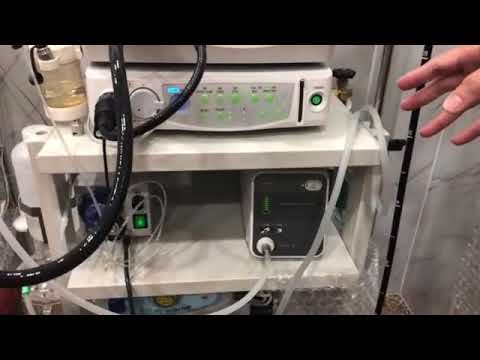The photograph, captured indoors, features a horizontally rectangular image framed by thin black borders at the top and bottom. Dominating the scene is a white, multi-tiered shelf displaying various pieces of interconnected medical equipment. Central to the image, on the top shelf, sits a white device adorned with light mint green buttons, a white dial on the left, and a red and green indicator light. This device is accompanied by several cords and tubes, including a thick black wire that could be a power cord. Adjacent to it is a component that resembles a battery pack. Below, on a middle shelf, lies another apparatus, a white and black box equipped with a tube, and a white box featuring a green and red light. To the far left of the shelves, a translucent container with a clear greenish liquid is visible, possibly part of a pumping system. In the upper right-hand corner of the image, a tan hand with splayed fingers and an extended thumb is seen reaching towards the equipment, adding a human element to the technical tableau.